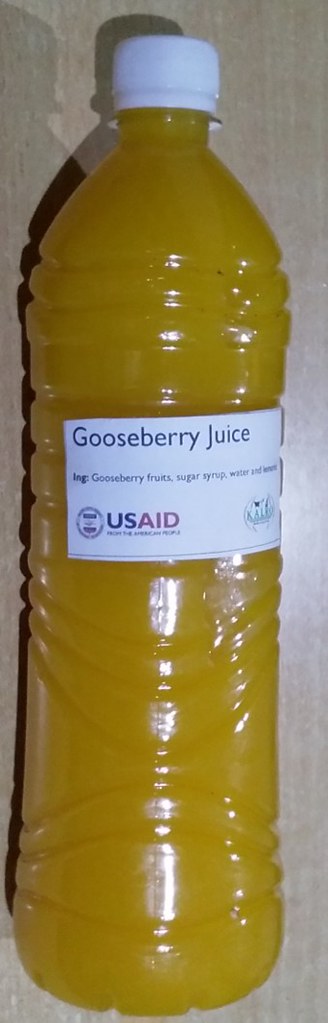Photograph of an orange-colored Gooseberry Juice beverage in a plastic bottle with a white cap. The bottle is resting on a blonde wooden surface, casting a gray shadow on the table. The front label is white with black font stating "Gooseberry Juice," while smaller black text below it mentions "USAID." To the side of the label, there is an icon featuring green coloring with a small navy mark above it. Light reflections can be seen on the plastic bottle, which appears slightly flimsy.